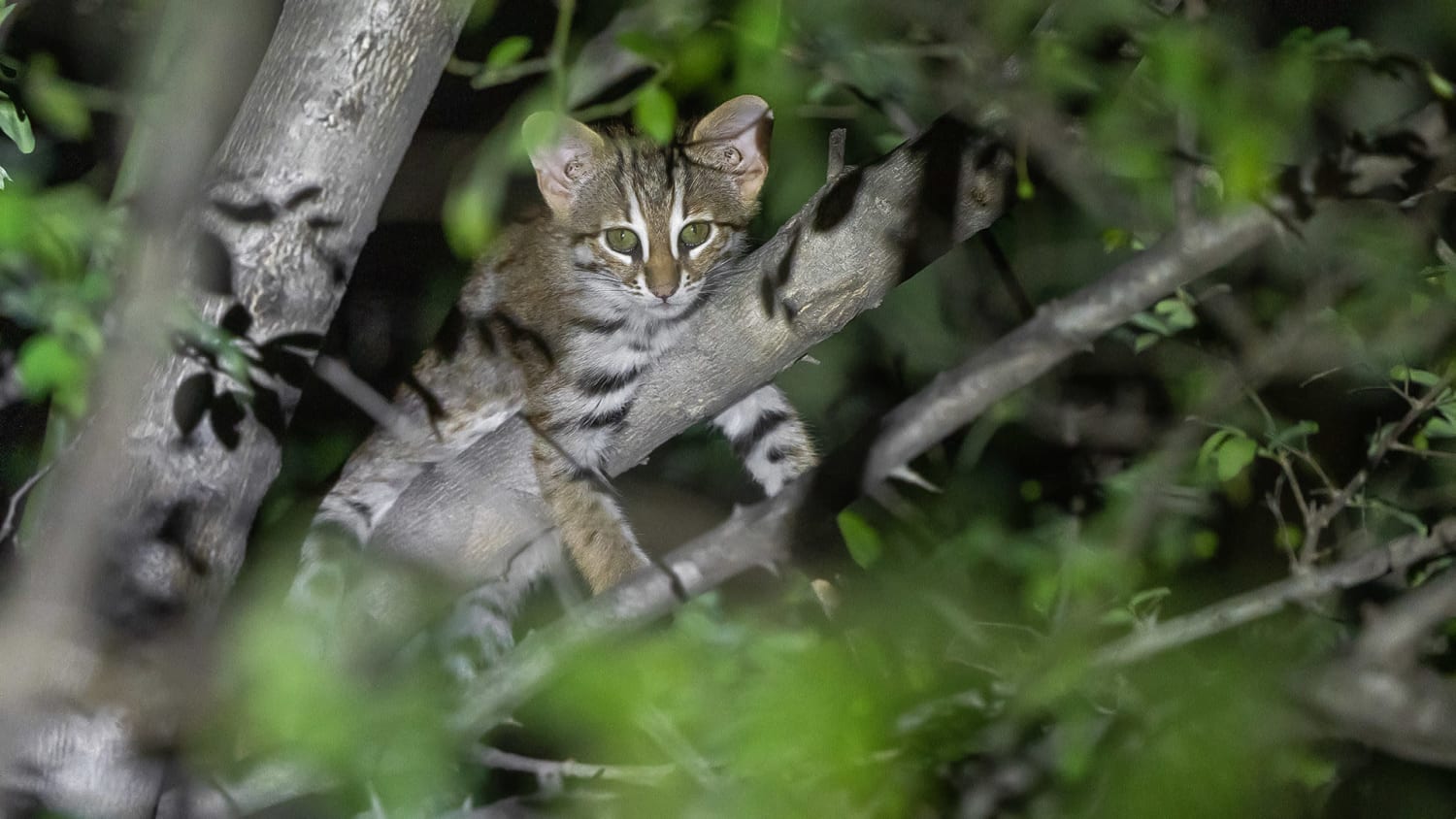A detailed nighttime photograph captures a small, striped kitten comfortably nestled on a branch in a tree. The cat, which has sizable ears and striking green eyes, gazes directly at the camera, illuminated by the flash. Its fur blends hues of gray, black, white, and subtle hints of gold, forming a tiger-like pattern. The surrounding leaves in the foreground are blurred, giving a sense of depth to the image. The scene indicates a nighttime outdoor setting, with at least five visible branches, among which the kitten is perched on one, its tiny paws adorably dangling.